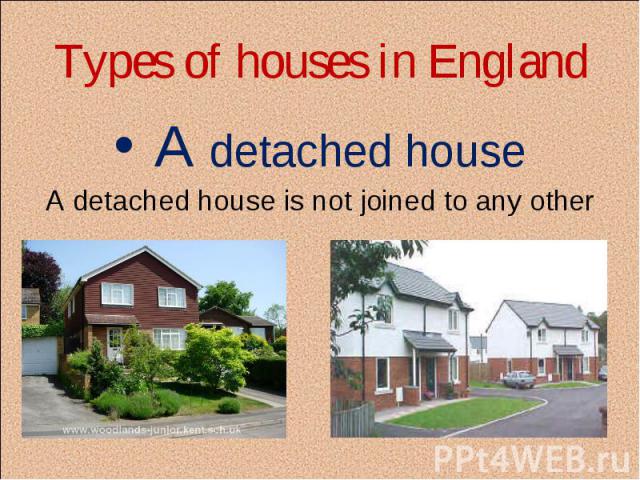The graphic, shaped as a horizontal rectangle in light tan, is titled "Types of Houses in England" in bold red letters centered at the top. Below, in blue font, it states, "A detached house is not joined to any other," and provides examples with two inset pictures. On the left, there is a red brick, two-story house with white windows, surrounded by lush green trees, shrubs, and a neatly landscaped yard. It features a paved driveway and a white garage on the side. On the right, two adjacent houses with white upper floors and red brick lower floors are shown, each with gray shingled roofs; a gray car is parked in front of this second set of houses. The entire layout suggests an informative piece about detached houses commonly found in England, possibly part of a larger real estate or educational presentation, emphasized by a discreet link to a Russian website in the bottom right corner.